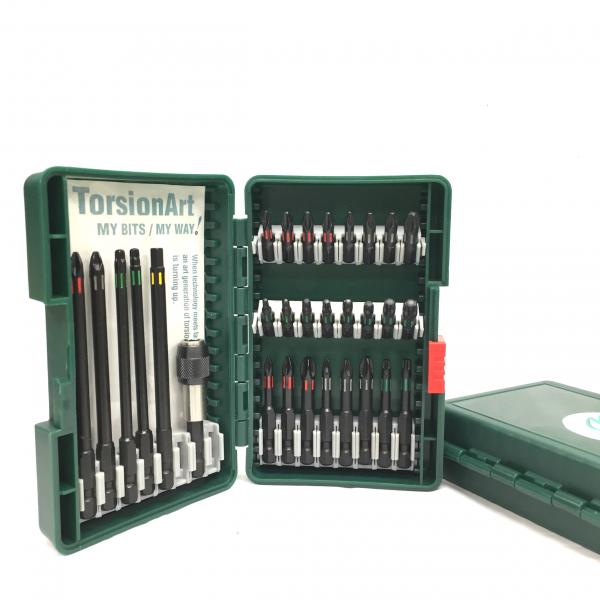This is a vibrant color photograph depicting a set of drill bits and screwdrivers displayed in two identical green plastic cases. The case on the left is open, showcasing the array of bits and tips meticulously organized within white holders. The open case reveals a neat arrangement: a row of long, predominantly black drill bits on the left, differing in head types, and sections of shorter bits and screwdriver tips, including several Phillips heads. Adjacent to the drill bits, three white strips securely hold additional rows of these various bits.

To the right of the open case, the second case remains closed, providing a clear contrast between the contents and the protective exterior. The cases feature an orange latch on the right-hand side, ensuring secure closure. Behind the bits inside the open case, a piece of white paper with green text reads, "Torsion Art, My Bits, My Way." The entire setup is photographed against a clean, white backdrop, emphasizing the tools' organization and design details.